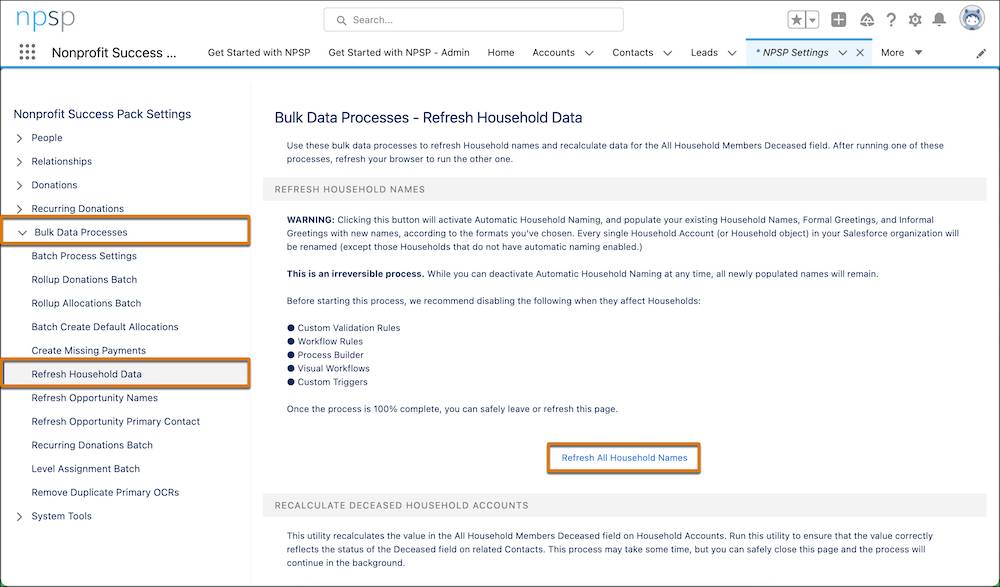**Descriptive Caption:**

The image is a screenshot from the NPSP (Nonprofit Success Pack) website, displayed on a computer monitor or laptop screen in landscape orientation. The website's name, "npsp," appears in the top left corner, with each letter in lowercase and in different colors: green, blue, dark blue, and light gray. Centrally positioned at the top of the page is a search bar with the word "search" inside it, accompanied by a magnifying glass icon to the left.

In the top right corner, there is a row of icons including a star, a drop-down arrow, a plus inside a box, an unidentified icon, a question mark, a settings (cog or gear) icon, and an alert (bell) icon. The extreme upper right corner features a user profile avatar, depicted as a circle containing a blue, cartoony caricature.

Moving back to the left side of the screen, there is a square composed of three rows of four dots, adjacent to the text "Nonprofit Success..." Further down, there are navigation options labeled as "Get Started with NPSP," "Get Started with NPSP Admin," "Home," "Accounts," "Contacts," "Leads," and "More," each with a drop-down arrow. Additionally, there is an option labeled "NPSP Settings," which has been clicked, highlighted by a blue tab with a matching thin blue line stretching across the screen beneath it.

On the left-hand side of the page, there is a column of clickable options under the header "Nonprofit Success Pack Settings." These options include "People," "Relationships," "Donations" (the precise text is slightly unclear due to small font size), "Recurring Donations," and "Bulk Data Processes." The "Bulk Data Processes" option is selected, indicated by a red rectangle outline and a down-pointing arrow, which reveals subheadings such as "Batch Process Settings," "Roll Up Donations Batch," "Roll Up Allocations Batch," "Batch Create Default Allocations," and "Create Missing Payments."

On the right side of the screen, the main display area shows content related to "Bulk Data Processes" with the heading "Refresh Household Data." Below the heading is a mix of sentences and bullet points in small font, and at the bottom of this area, there is a red rectangle containing a button labeled "Refresh All Household Names."